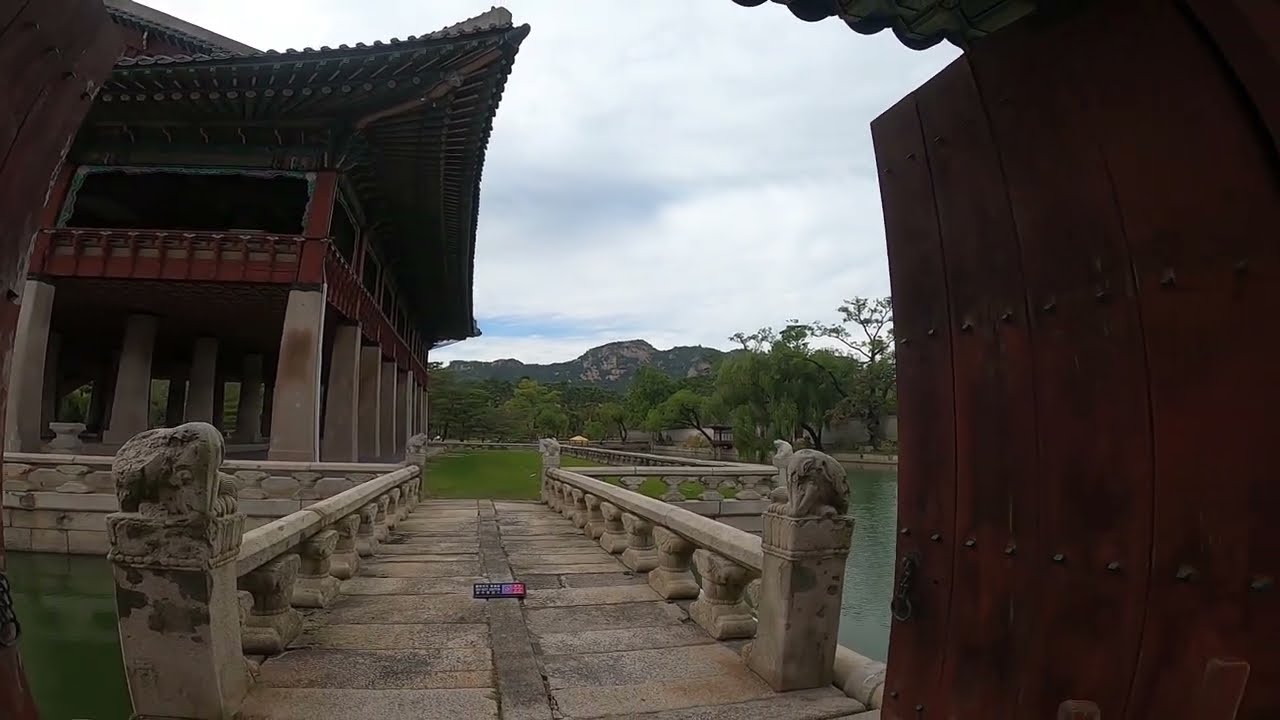This image captures the entrance to a historic East Asian temple complex with distinctive traditional architectural features. The scene is set outdoors on a partly cloudy day with a touch of blue sky peeking through. The focal point is an ancient stone pathway bordered by robust stone partitions and concrete railings. On both sides of the path are impressive pillars, possibly adorned with carved animals.

To the right, a reddish-brown wooden wall with vertical planks, potentially a door, is visible. Above this wall, part of the temple roof structure, painted in rich red and green hues, comes into view, consistent with traditional Chinese or Japanese architectural styles. On the left side, another temple structure stands atop high gray geometric stone pillars, featuring intricate wooden overhangs and dark brown-red wooden elements.

The path crosses over a serene body of water, which glistens with shades of greenish-blue. This water appears tranquil and almost still, creating a reflective surface that enhances the visual depth of the image. Surrounding the temple complex is a lush landscape with greenery, including distinctive weeping willows and other trees. In the background, a striking mountain range with a rocky formation stretches across the horizon, completing the picturesque scene.